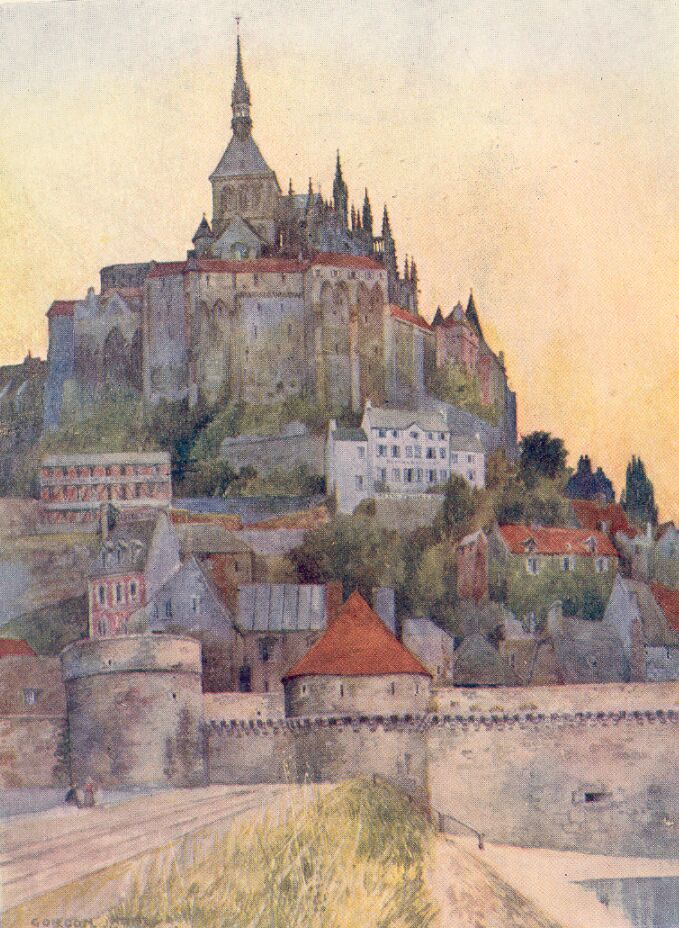The painting vividly illustrates a grand white castle perched high on a hilltop, characterized by striking red roofs with several towering points, signifying its majestic and fortified nature. Below the castle, a cluster of smaller buildings with similar castle-like architecture sprawls across the landscape, nestled within the contours of the hill. In the very foreground, a stretch of verdant green grass is bordered by a grey stone wall, possibly serving as a barrier or boundary. 

A roadway meanders up the hill towards the main entrance of the village, implying a security checkpoint or gate, lending an air of guarded exclusivity. Beyond this bustling settlement lies a panoramic view that merges seamlessly into a pastel sky. The sky transitions beautifully from soft blue at the top to a glowing pink-orange hue near the horizon, suggesting either the dawn of a new day or the gentle retreat of the sun into dusk. To the right of the scene, a white-green strip of land adds an intriguing natural element, possibly a ditch or a steep cliff, enhancing the dramatic and imposing atmosphere of the location.